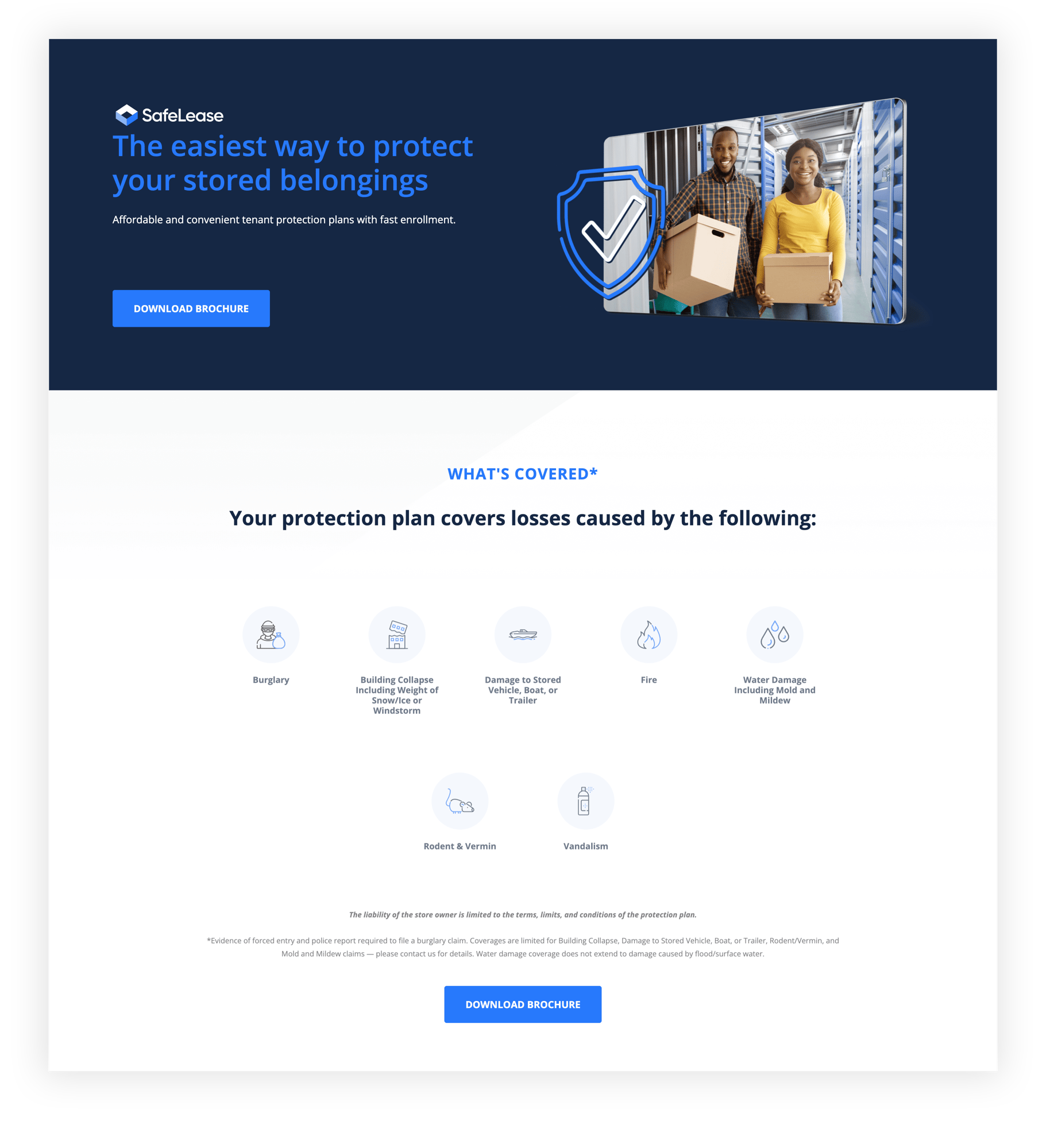Caption: 

"In a brightly lit storage facility, a young Black couple stands in a narrow hallway between rows of blue corrugated gates, each holding a box. Their smiles radiate excitement as they utilize Safelease, the easiest way to protect their stored belongings. The scene, set within a personal storage environment, is accompanied by a shield with a check mark symbolizing security and peace of mind. Above the image, a large 'Download Brochure' button invites viewers to learn more, set against a navy blue background that transitions to white further down. Text details the comprehensive coverage provided by Safelease, including protection against burglary, building collapse, vehicle damage, fire, water damage, rodents, and vandalism. Another download button is placed near the bottom, emphasizing accessible information. Safelease offers a reliable insurance plan, ensuring users can store their items with confidence and ease."